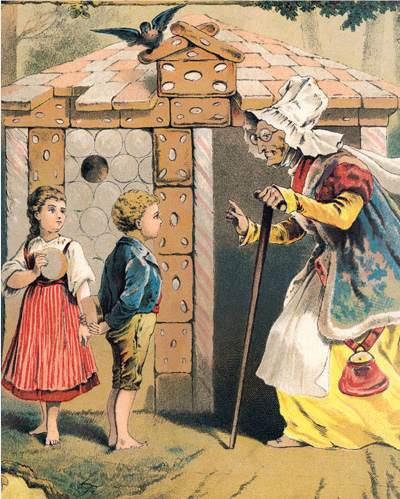This detailed drawing portrays a scene reminiscent of Hansel and Gretel. On the right side of the image stands an old woman with witch-like features, characterized by her very pointed chin and deeply wrinkled face. She wears a tall white bonnet that drapes over her head and round glasses. The old woman is dressed in a long blue robe, accented with a white apron and a yellow underskirt. A white scarf trails behind her, and in her left hand, she grips a long cane that extends to the dirt ground.

To her left are two young children, appearing to be around nine or ten years old. The boy stands closer to the woman, sporting blonde hair, a blue jacket, and yellow knee-length pants. He is barefoot, standing on the bare ground. Behind him is a girl of the same age, also with blonde hair, dressed in a white blouse paired with a red dress that extends below her knees. She, too, is barefoot and holding a round carton.

The background features a house with distinctive architecture: the walls are constructed from brown and gray cement blocks, and the roof is made of rounded wood and bricks. At the very top of the house, a brown section resembling a bird's nest holds a black bird with its wings extended. In the upper right corner of the picture, the tree branches hang down, adding to the whimsical and slightly eerie atmosphere of the scene.